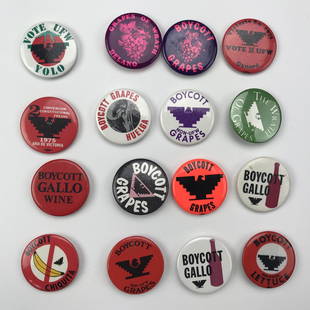The image showcases a collection of 16 circular buttons arranged in a 4x4 grid on a white background. Each button is unique, but many share common themes related to activism and voting. Most prominently, several buttons feature slogans such as "Boycott Grapes," "Boycott Gallo," and "Boycott Lettuce," accompanied by various designs. One button stands out with "Boycott Bananas" printed on it, suggesting a potentially humorous twist. The buttons also include messages promoting voting for the United Farm Workers (UFW), with symbols like eagles and text in different colors including red, black, green, and purple. Notable among them, the top left button is white with a red center and a black bird, inscribed with "Vote UFW Volo." The assortment of colors and designs across the rows contributes to a visually striking and historically rich image, indicative of past activism efforts.